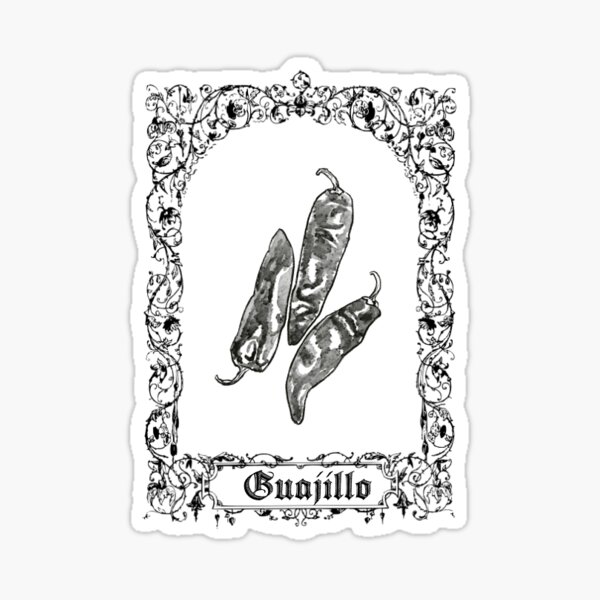This detailed black and white drawing centers on three guajillo peppers, meticulously illustrated in shades of gray. The composition features one pepper with its stem pointing downwards on the far left, a second pepper with its stem pointing upwards in the middle, and a third pepper positioned slightly tilted to the two o'clock direction with its stem also facing upwards. Encasing these peppers is an ornate filigree border composed of intertwining vines and flowers, creating an elegant arch around the image. The background is stark white, presenting a clean contrast against the intricate details. At the bottom of the drawing, 'Guajillo' is prominently displayed in a gothic, jagged script, enclosed within a boxed area that interrupts the vine border. The edges of the image resemble aged, scalloped paper, contributing to its vintage, decorative allure—perfect for adding a rustic charm to a kitchen wall.